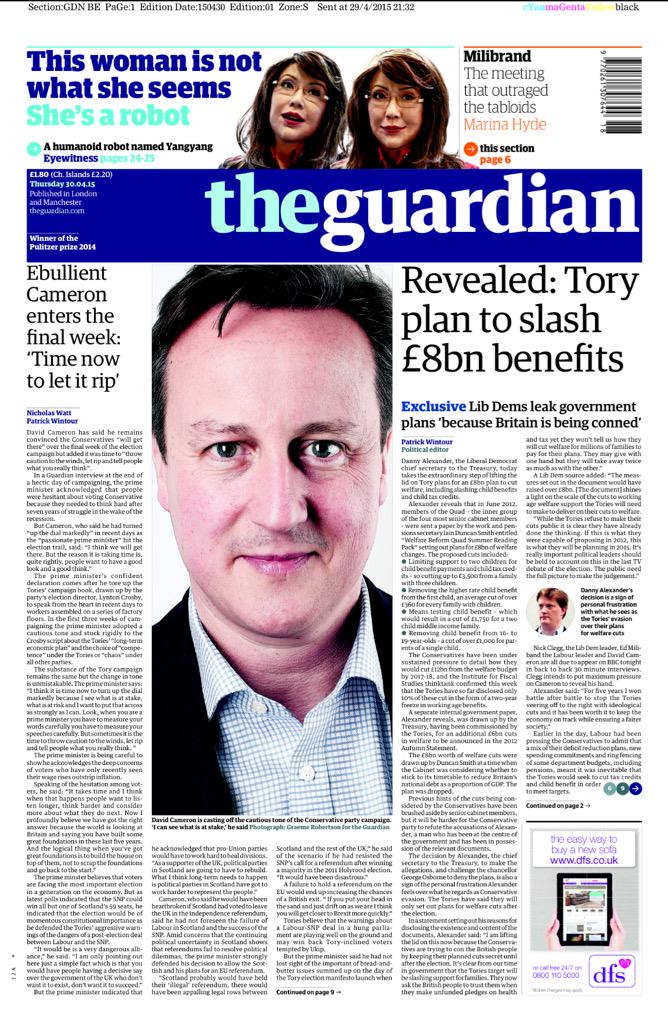The image features two side-by-side pictures of a woman with brown hair, glasses, and dark red lipstick. At the top of the image, a white border contains text that reads, "This woman is not what she seems - she's a robot." The woman is identified as a humanoid robot named "Vangang." To the right of the images, additional text states, "Mil-Milbrand: The meeting that outraged the tabloids" by Marina Hyde. A barcode is also present on the right side of the image.

Below the pictures and the initial text, there is a dark blue box with "The Guardian" written on it. To the left of this box, there is some small and blurry text that appears to be in Chinese, although it cannot be read clearly.

Underneath the blue box, a headline reads, "Ebullient Cameron enters the final week: time now to let it rip." Next to this headline, on the right side of the image, there is a large photograph of a man with black hair, brown eyes, and a light complexion. He is wearing a shirt with a collar featuring white and blue squares and a black suit jacket.

To the right and left of the man's picture, there are several paragraphs of text, but the text is too small to read.